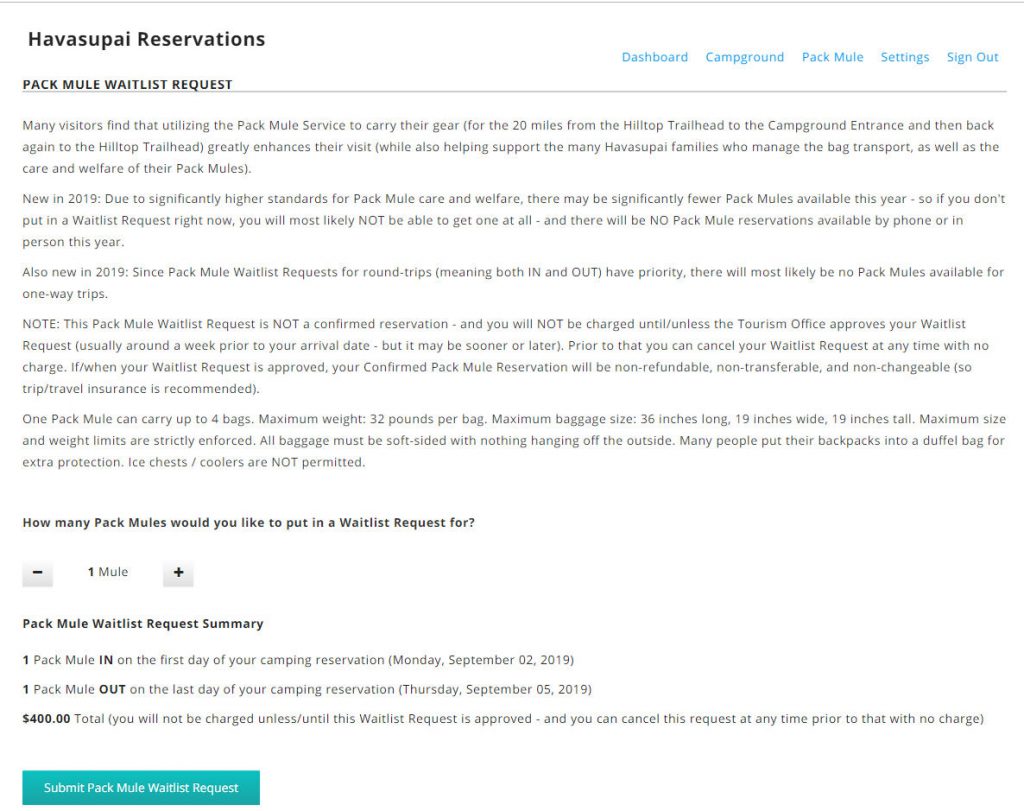The image showcases a detailed web page layout for requesting a pack mule service to transport camping gear. At the top right of the page, there are navigation buttons labeled "Dashboard," "Campground," "Pack Mule," "Settings," and "Sign Out," which are highlighted in blue. On the left side, a heading reads, "Have a Supply Reservation," followed by an informative article titled "Pack Mule Waitlist Request."

The article states that many visitors benefit from the pack mule service, which carries their gear along the 20-mile journey from the Hilltop Trailhead to the Campground Entrance and vice versa. This service greatly enhances their camping experience and supports the families who manage the mules. However, new regulations introduced in 2019 to ensure higher standards of care for the mules have reduced their availability. Therefore, making a waitlist request immediately is advised. 

Key points include:
- A significant reduction in pack mules available, urging early waitlist requests.
- Reservations are neither available by phone nor in person this year.
- Priority is given to round-trip requests, with limited availability for one-way trips.

Important notes:
- Waitlist requests are not confirmed reservations. They are only charged upon approval by the tourism office, typically a week before arrival but potentially sooner or later.
- You can cancel waitlist requests at any time before approval without any charge. Once confirmed, reservations are non-refundable, non-transferable, and non-changeable. Travel insurance is recommended.
- A pack mule can carry up to 4 bags, each not exceeding 32 pounds and 36x9x9 inches. Ice chests or coolers are prohibited, and all baggage must be securely packed.
  
The page features interactive elements, including plus and minus signs to adjust the number of pack mules requested. At the bottom, the "Pack Mule Waitlist Request Summary" outlines a sample request: one mule in on the first day of camping (Monday, September 2019), and one mule out on the last day (Thursday, May 5, 2019). The $400 fee will only be charged upon approval, and cancellation is free before that point.

A green "Submit Mule Waitlist Request" button is positioned at the bottom left, ready for the final submission.